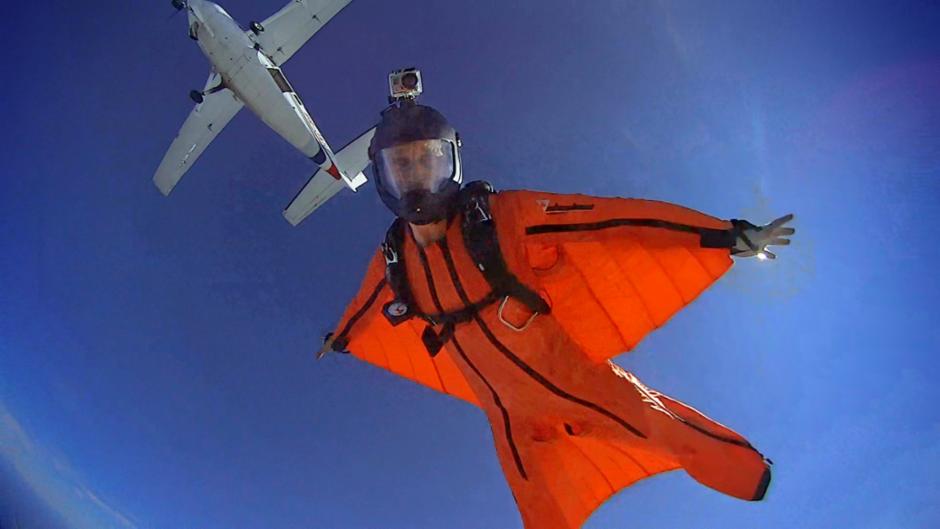This photograph captures a thrilling moment of a man skydiving from a small white airplane that is visible above him. The skydiver, who appears male, is the central figure in the image, donned in a bright orange wingsuit reminiscent of a flying squirrel or a bat, with fabric flaps extending from his arms to his body, allowing him to control his descent. He is equipped with a black helmet featuring a clear face shield, and a GoPro camera mounted on top, suggesting a similar setup for the photographer, possibly attached to their head. The sky around them is a vivid blue, nearly cloudless, with the Sun partially obscured by the skydiver's outstretched left hand. The perspective of the photograph is from below, looking up at the skydiver, highlighting the exhilarating altitude and the airplane he just exited, emphasizing the sheer height and freedom of the jump.